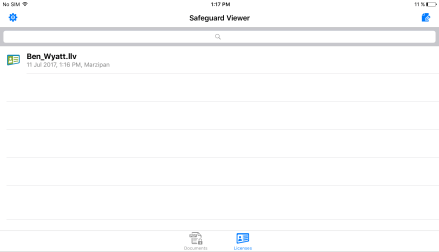This image is a minimalistic digital interface with various icons and text elements. In the upper left-hand corner, there is an unreadable text with a blue deer icon beneath it. Centered on the image is the time, displayed as 1:17 p.m., with the word "safeguard" written underneath. To the right, there is an indication of an 11% battery level alongside a battery icon. Below this is an unfamiliar blue icon.

A gray rectangular search box, outlined with a thick gray line, features a magnifying glass icon in its center. Underneath the search box, there appears to be a small card icon with a depiction of a person and illegible text to its right. The bold black name "Ben_Wyatt_THB" is prominent, though the text beneath it is unreadable.

Following this are six very thin gray lines, evenly spaced. To the lower right are indistinct gray and blue icons, and a thicker horizontal gray line runs at the bottom of the image.